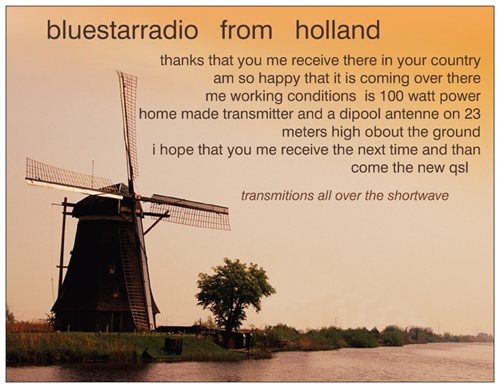The image appears to be a screenshot reminiscent of a Facebook post, featuring a photograph with an overlay of some text. The photo depicts a brown windmill near a lakeside, accompanied by a tree, amidst a background of reflective water and sky. The entire scene is tinted with an orangish hue, suggesting the time of day might be early morning or late evening.

The text overlaid on the sky reads: “Blue Star Radio from Holland. Thanks that you may receive there in your country. I'm so happy that it is coming over there. Me working conditions is 100 watt power, homemade transmitter, and a deep pool antenna 23 meters high about the ground. I hope that you, me, receive the next time and then come the new QSL. Transmissions all over the shortwave.” 

The grammar and spelling indicate that English is likely not the first language of the person who posted this, as evidenced by phrases like “me working conditions" and "receive you, me.” This suggests they are sharing their joy about their radio station, Blue Star Radio, reaching listeners overseas using modest equipment.